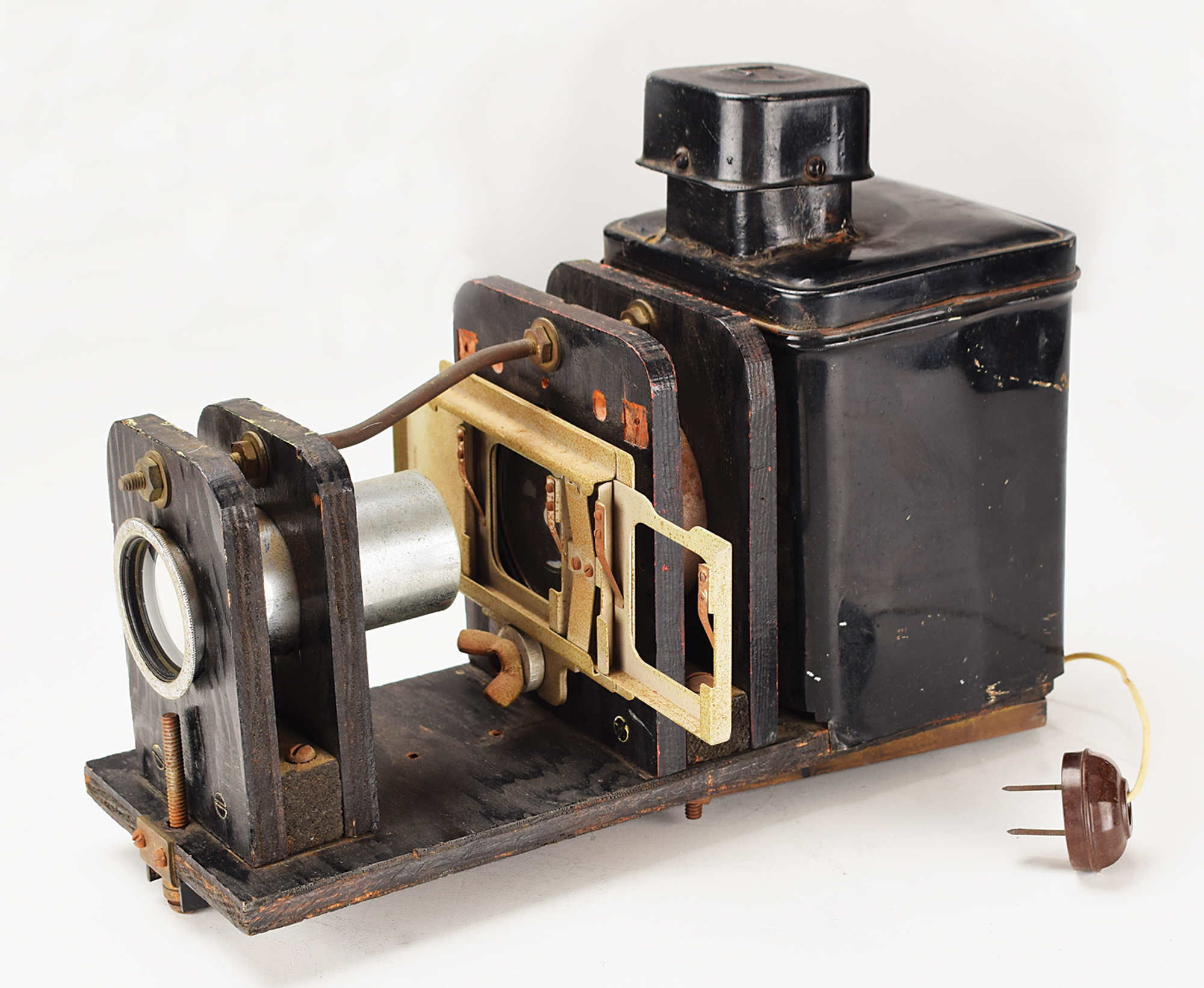The image depicts an antique slide projector, reminiscent of early 20th-century designs. The body of the projector is primarily black and constructed from metal at the back, which includes a cylindrical component and a light brown opening. The front section, facing left in the image, is characterized by four black wooden boards. The central feature on the front is a circular lens opening, bordered by a silver metal ring. This classic device, resembling a squat metal box with a chimney-like top, is mounted on a wooden plank. A distinctive yellow wire links the bottom right of the projector to a socket, which is not plugged in. The overall aesthetic and materials suggest that this projector was used during the era of early black-and-white films, likely from the 1920s.